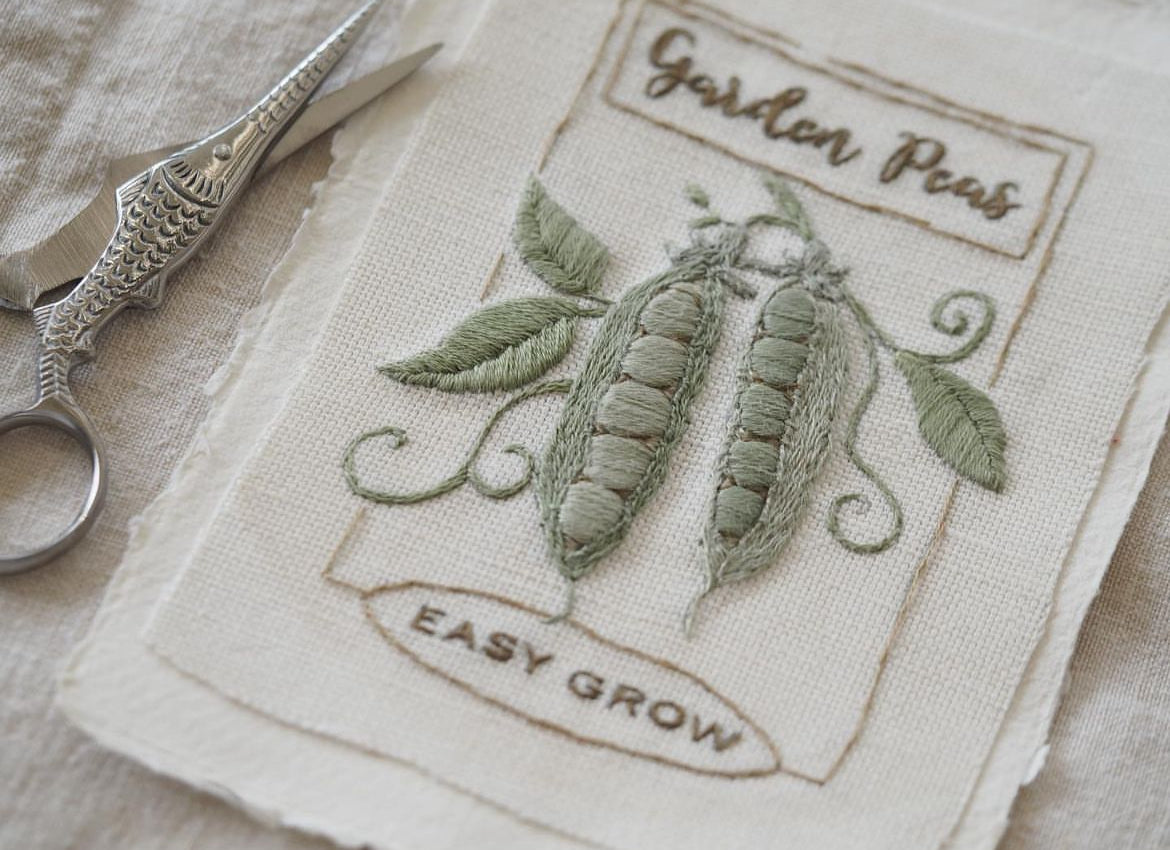This black and white photograph features a richly detailed piece of embroidery, presenting an intricate depiction of a vintage garden pea packet. The embroidered cloth, resembling IATA fabric, displays "Garden Peas" prominently at the top in brown thread. The center features two long pea pods, each containing five peas, rendered in light green thread with delicate leaf and stem details extending from them. At the bottom, the words "Easy Grow" are meticulously stitched within a capsule-shaped outline. The craftsmanship on the embroidery is impeccable, suggesting the colors—though unseen in the monochrome image—would be vivid and striking.

Lying diagonally on a cream to gray, linen-like surface, the embroidery is accompanied by a pair of ornate, probably antique, scissors positioned on its left. These small, silver scissors boast an intricate fish motif on one of the handles, reminiscent of a swordfish. The detailed and decorative design of the scissors implies rarity as such elegance is seldom found in contemporary designs. The interplay of textures and details, from the stitched fabric to the ornate scissors, makes for a visually captivating scene that evokes a sense of nostalgia and admiration for detailed handiwork.